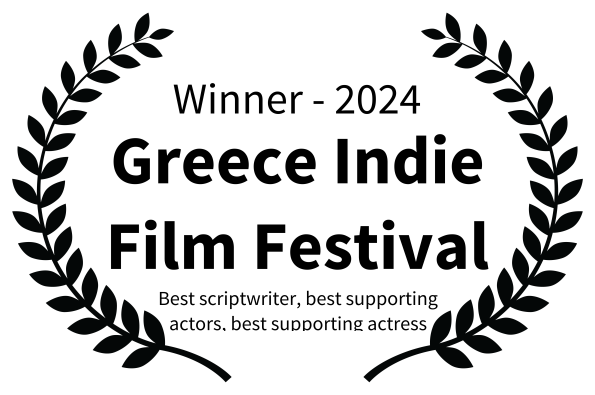The image is a black and white banner for a web page, designed to commemorate the Winter 2024 Greece Indie Film Festival and announce award winners. The background is white, and the text and graphics are rendered in black. Symmetrical vine-like ferns with smaller leaves grow along the left and right edges, arching outward to create a parenthesis-like frame around the central text. In bold letters, the banner announces "WINTER 2024 GREECE INDIE FILM FESTIVAL." Beneath this, in smaller font, it lists the awards: "Best Script Writer, Best Supporting Actors, Best Supporting Actress." The design is simple and uncluttered, with the ferns not connecting at the top or bottom, leaving space around the central text. The section mentioning "Supporting Actress" appears slightly cut off, suggesting a portion of the banner may be missing or imperfectly rendered.